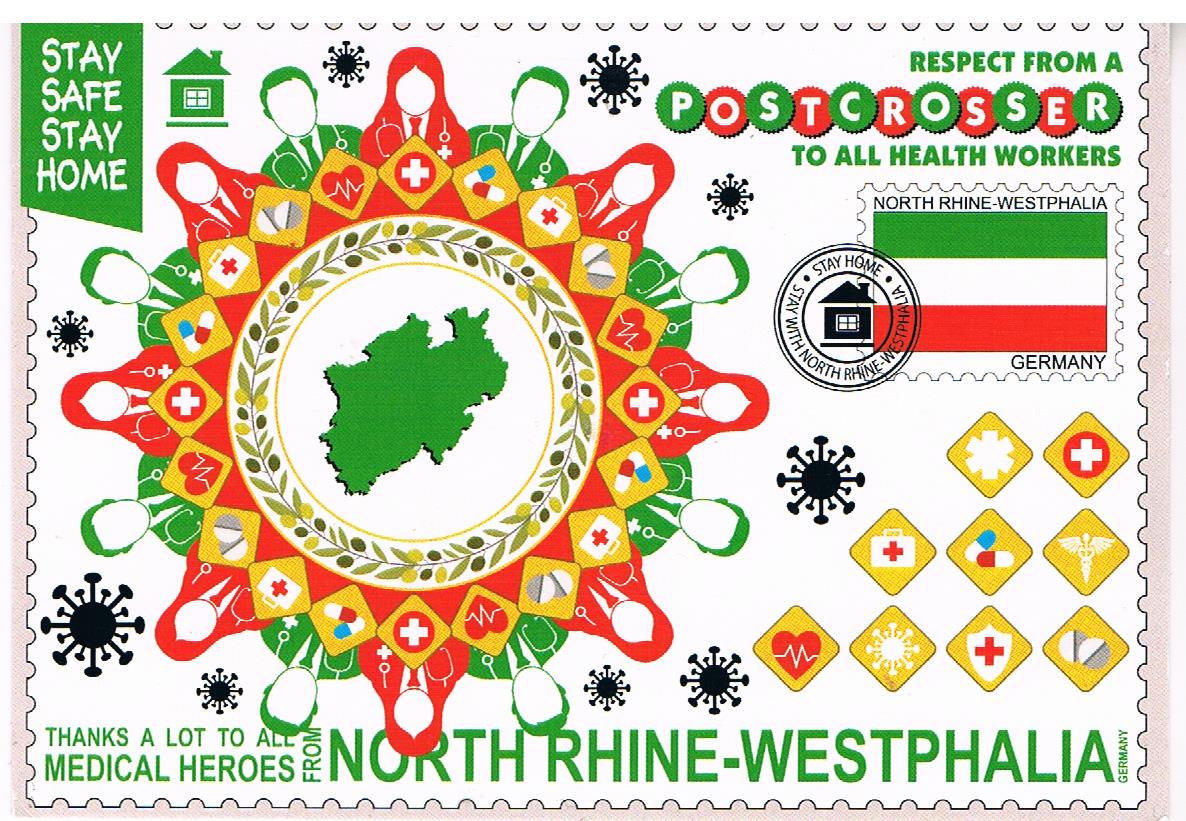This image features a detailed stamp from North Rhine-Westphalia, Germany, designed as a tribute to healthcare workers during the COVID-19 pandemic. The stamp's border has the characteristic serrated edging, and at the upper left corner, a green skewed rectangle with the white text "Stay safe, stay home" is prominently displayed next to a small green house icon. Central to the stamp is a circular motif depicting an aerial view of North Rhine-Westphalia, surrounded by alternating red and green line-drawn silhouettes of healthcare professionals wearing stethoscopes. Scattered around this central image are various medical symbols such as red and white crosses, a heart symbol, and pills, integrated into diamond-shaped areas.

In the upper right, the text "Respect from a post-crosser to all health workers" is presented with each letter contained within alternating red and green circles. Directly beneath this text, a flag of North Rhine-Westphalia with horizontal stripes of green, white, and red is visible. At the very bottom of the stamp, the message "Thanks a lot to all medical heroes from North Rhine-Westphalia, Germany" is inscribed, emphasizing gratitude towards medical professionals. Together, these elements create a visually rich and heartfelt tribute to the extraordinary efforts of healthcare workers during the pandemic.